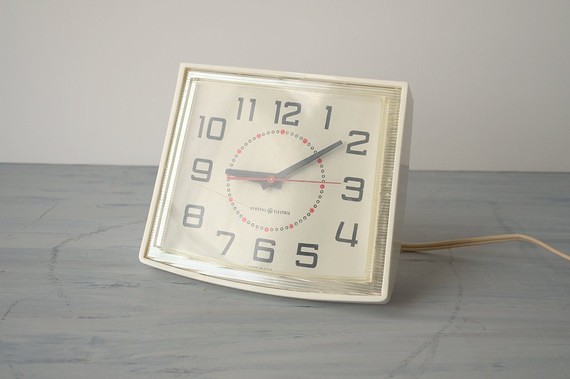The image shows an older, rectangular analog clock placed on a gray wooden-textured desk. The clock is predominantly white with a slightly off-white, almost grayish face. It features black hour numbers, black minute ticks, and a dotted circle for the hour markers, which are red. The clock hands include a black hour hand, a black minute hand, and a thin red second hand. The clock appears to be reading 9:09. Additionally, the device is connected with a brownish-tan power cord that extends towards the left. The background features a white wall, and there is some glare on the clock face, likely from the photographer's light source.